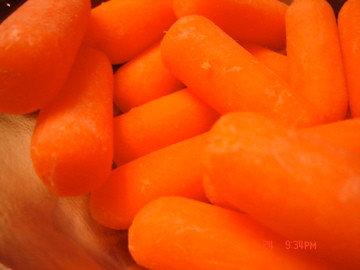The image is an extreme close-up of over a dozen baby carrots, all orange and oblong, with cylindrical shapes and rounded ends. These carrots are piled haphazardly onto a surface that is difficult to identify— it might be a hand, a napkin, or a bowl. Notably, the carrots lack any wetness or condensation, appearing distinctly dry and uneaten. Each carrot is roughly the same size, epitomizing the uniformity and appeal of baby carrots. The image includes a timestamp reading 935 p.m. in red, located in the bottom right-hand corner. The objects range from the near lower right of the frame up to the top and stretch across to both the top and bottom right edges of the image, which has a cramped, horizontal format.